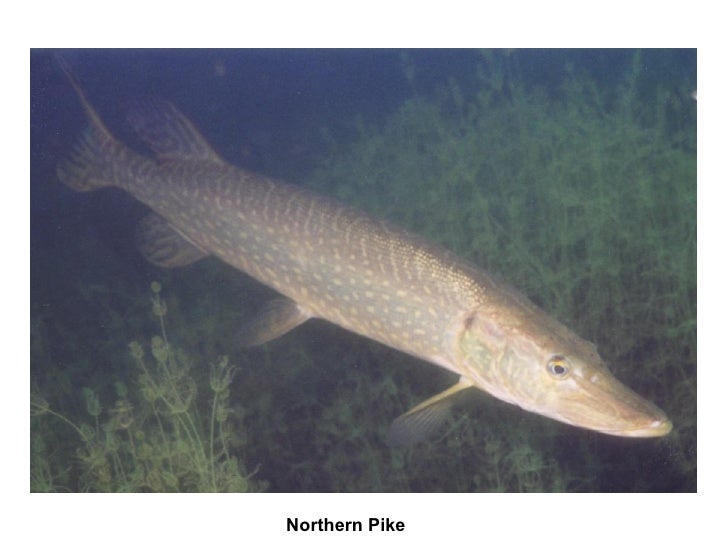In this horizontal photograph of a Northern Pike, the fish is swimming in dark blue water surrounded by green plants growing both in the foreground and background. The fish is long with spots and stripes on its body, showcasing a gradient of colors from a lighter grayish-brown at the head to a darker bluish-brown towards the tail. The long mouth extends in front of its black eye, which is positioned near the lower right-hand corner of the image. Four fins are visible: three on one side and one on the other, along with its tail. The greenery near the dorsal fin adds to the intricate details of the underwater scene. The words "Northern Pike" are written in plain black text at the bottom of the image. Some darkness adds depth to the upper left-hand corner of this image, which is not very high in resolution but still clearly displays the distinct features of the fish.